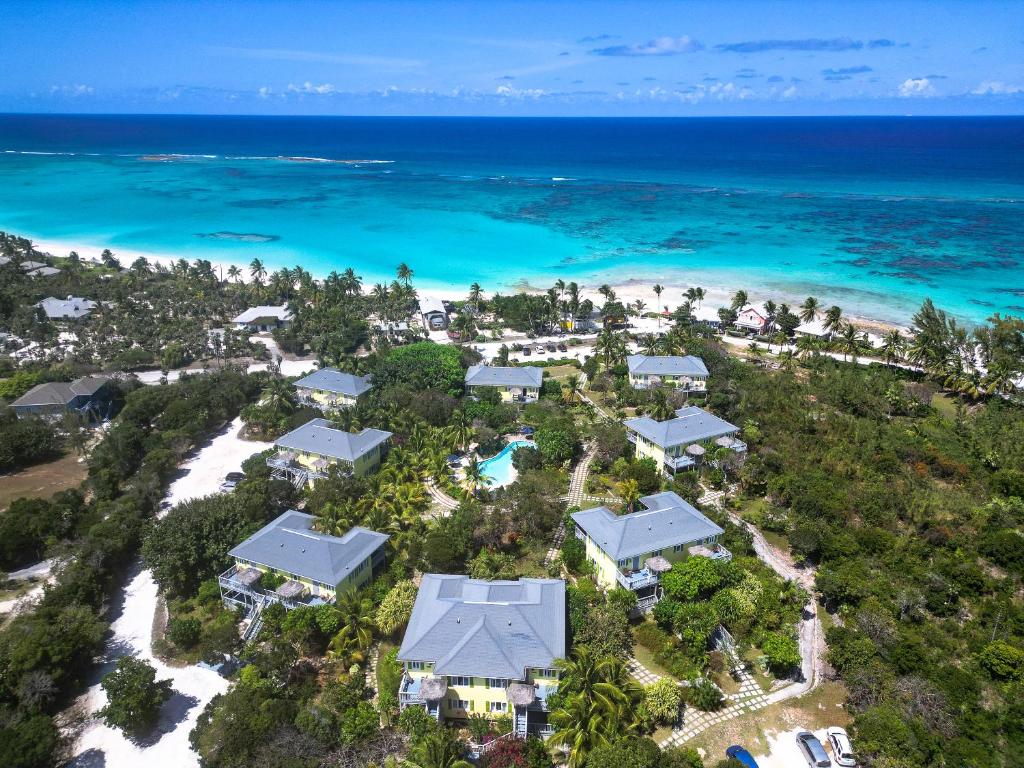This aerial photograph captures a tropical coastal community, possibly a beach resort or a living community, surrounded by lush greenery and abundant palm trees. Eight nearly identical yellow-painted homes with silver-gray roofs are organized around a central shared pool, suggesting a condominium or vacation rental setup. Pathways and small roads connect the buildings, with three small vehicles—white, silver, and dark-colored—visible in the bottom right corner of the image. The community is nestled beside a picturesque white sand beach, leading to a shallow, clear blue section of water speckled with coral and rocks before the ocean deepens to a darker shade of blue. A few clouds dot the sky, adding to the serene, inviting atmosphere of this tropical paradise.